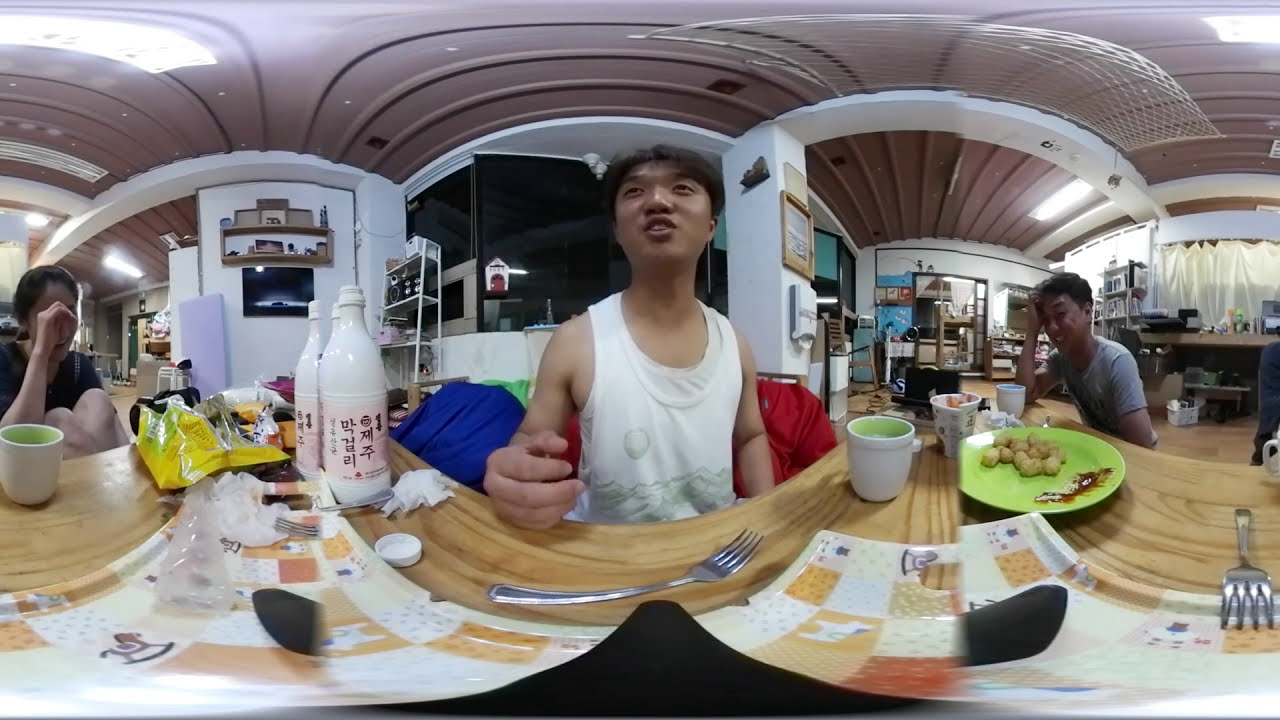The photograph captures a lively, panorama-like scene featuring three young individuals, possibly in their twenties, centered around a lightwood counter that seems to be part of a casual setting, potentially a restaurant or a communal dining area. In the center sits an Asian male wearing a white muscle shirt decorated with a green mountain design. Positioned in front of him on the counter are a fork and a mug filled with green liquid, possibly matcha tea. To his left is a young white woman, also enjoying a similar green beverage from a white mug. Her right hand is raised to her face, perhaps wiping away tears of laughter or hiding her giggles. On the right, another Asian male, dressed in a gray shirt, holds his right hand near his temple as if steadying himself or focusing. His plate, adorned with tater tots and a dollop of ketchup, adds to the casual dining vibe. Behind them, various white bottles with Korean text and other snacks suggest a Korean household or a dining venue. The background reveals white walls with artworks, creating a cozy yet slightly cluttered atmosphere, hinting that it could be a storage area, workplace, or relaxed communal space, likely lit during the evening as suggested by the dark ambiance and ceiling lights. All three appear to be enjoying a casual, laughter-filled gathering amidst a backdrop of cultural decor and everyday items.